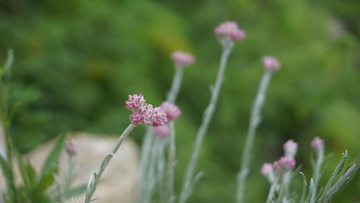This photograph captures a field where the main focus is a cluster of delicate flowers with pink and purple hues atop long, green stems. The primary flower, positioned slightly to the left, stands out distinctly, revealing its white-tipped petals. The background is intentionally blurred, highlighting the lush greenery and numerous similar flowers, which appear softer and less defined. To the right, other tall flowers blend into the vivid green backdrop of bushes and vegetation. A notable feature in the foreground is a large, light gray rock situated on the left corner, adding contrast to the scene's predominantly floral composition. The entire image evokes a serene, natural setting, devoid of human presence or animals.